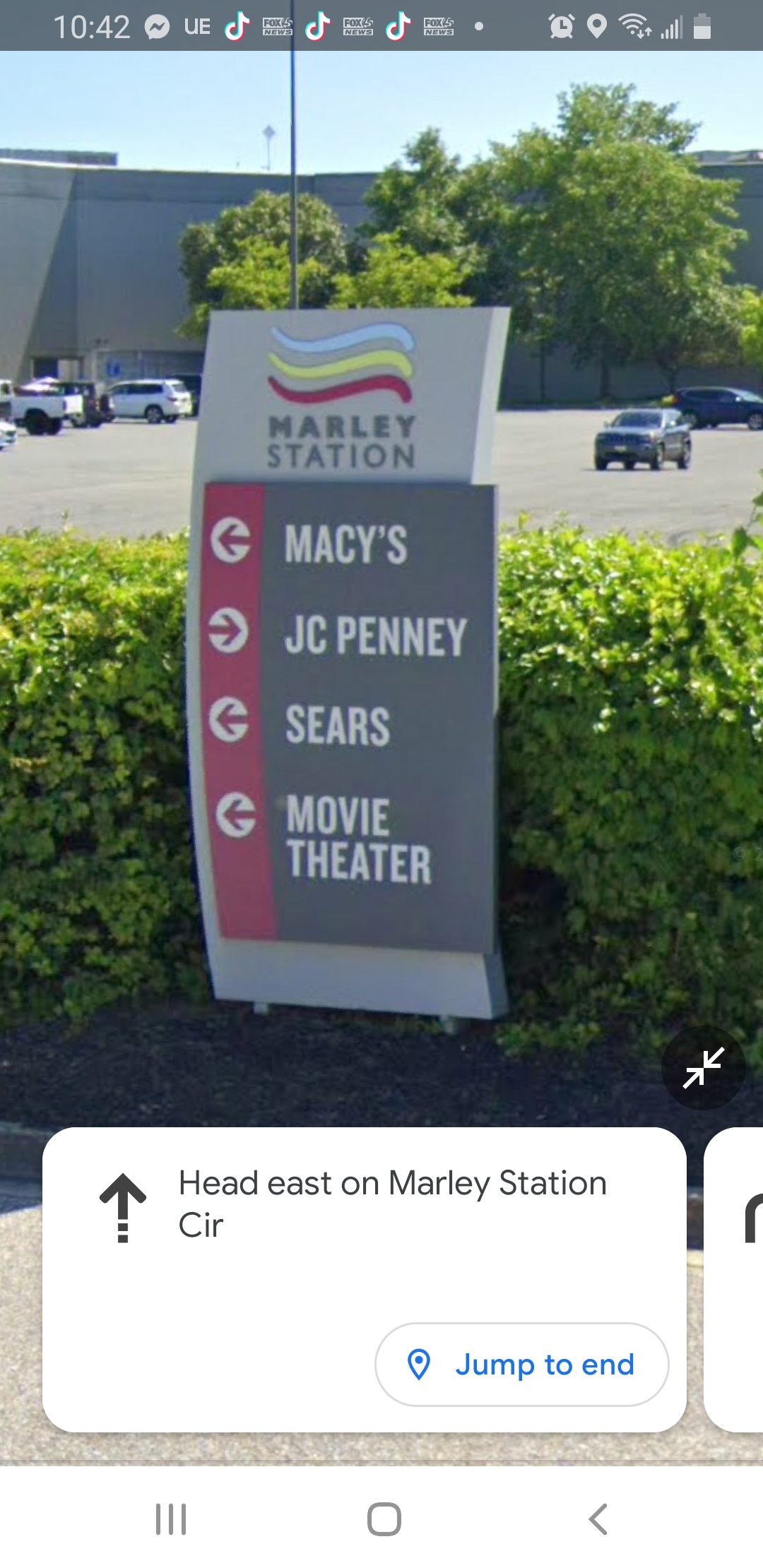The image depicted is a screenshot from a cell phone, showcasing a navigation app open and providing directions. At the top of the screen, there's a taskbar displaying the time as 10:42, various notification icons, an alarm clock symbol, a location tracking symbol, full Wi-Fi and mobile signals, and a battery level at half. Below this taskbar, there's a photograph showing a section of Marley Station Mall. The scene in the photograph includes a sign labeled "Marley Station," indicating directions to various stores and facilities within the mall: Macy's, Sears, and a movie theater all to the left, and JCPenney to the right. The sign is positioned in front of a well-maintained hedge, with a large, relatively empty parking lot visible in the background containing fewer than ten cars. Beyond the lot, additional trees can be seen near the mall building, which has a stone-colored exterior. Below the photograph, a white text bubble in the navigation app instructs to "head east on Marley Station Circle," with an option to "jump to the end" of the directions. The parking lot surface is described as a grayish asphalt.